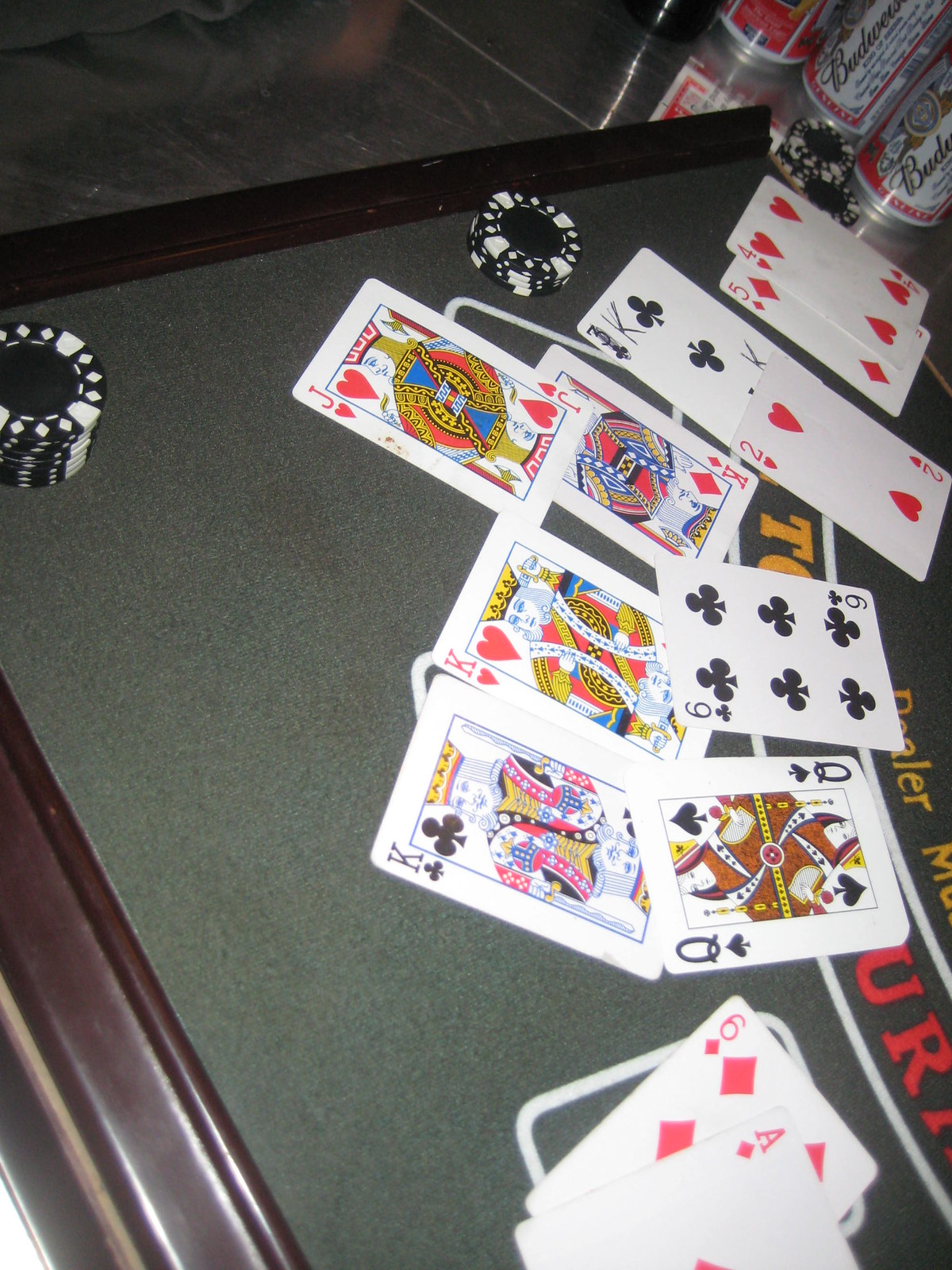This indoor photograph captures a lively poker game in progress on a wooden-style table with green felt. Positioned in the upper right corner of the image, several Budweiser beer cans suggest a casual and festive atmosphere. The table features a distinctive gray tile floor beneath it. Scattered across the table are black poker chips adorned with white designs on their edges and a variety of playing cards. The visible cards include the Four of Hearts, Five of Diamonds, Two of Hearts, King of Clubs, Jack of Hearts, King of Diamonds, Six of Clubs, King of Hearts, King of Clubs, Queen of Spades, and Six of Diamonds. The scene suggests an intense and engaging round of poker with participants likely enjoying both the game and their beverages.